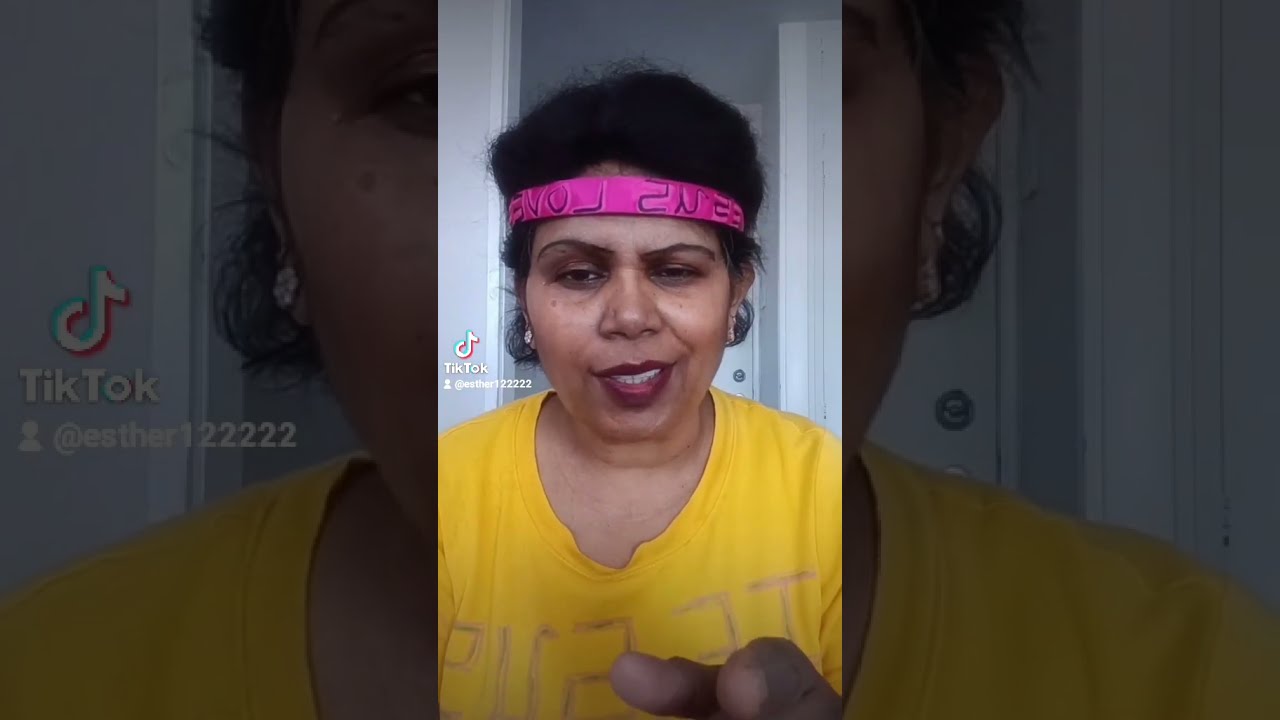The image is a screenshot of a TikTok video featuring a middle-aged woman with short dark hair pulled up. She's wearing a pink, rolled-up bandana around her forehead that has some writing on it, including the word "Love." She has small, flower-shaped, clear-stoned earrings in her ears and is dressed in a yellow t-shirt with some writing on it. The woman is partially smiling with a smirk and is pointing forward. The setting includes white walls and a white door in the background.

The image composition centers around a focused and highlighted vertical rectangle in the middle of the larger horizontal rectangle, creating a "picture within a picture" effect. To the left of her face is the TikTok logo with the handle @Esther122222. The overall colors in the image include hot pink, yellow, brown, beige, tan, black, dark red, white, and gray. The photograph includes framing on both the left and right sides, further emphasizing the central focus on the woman.